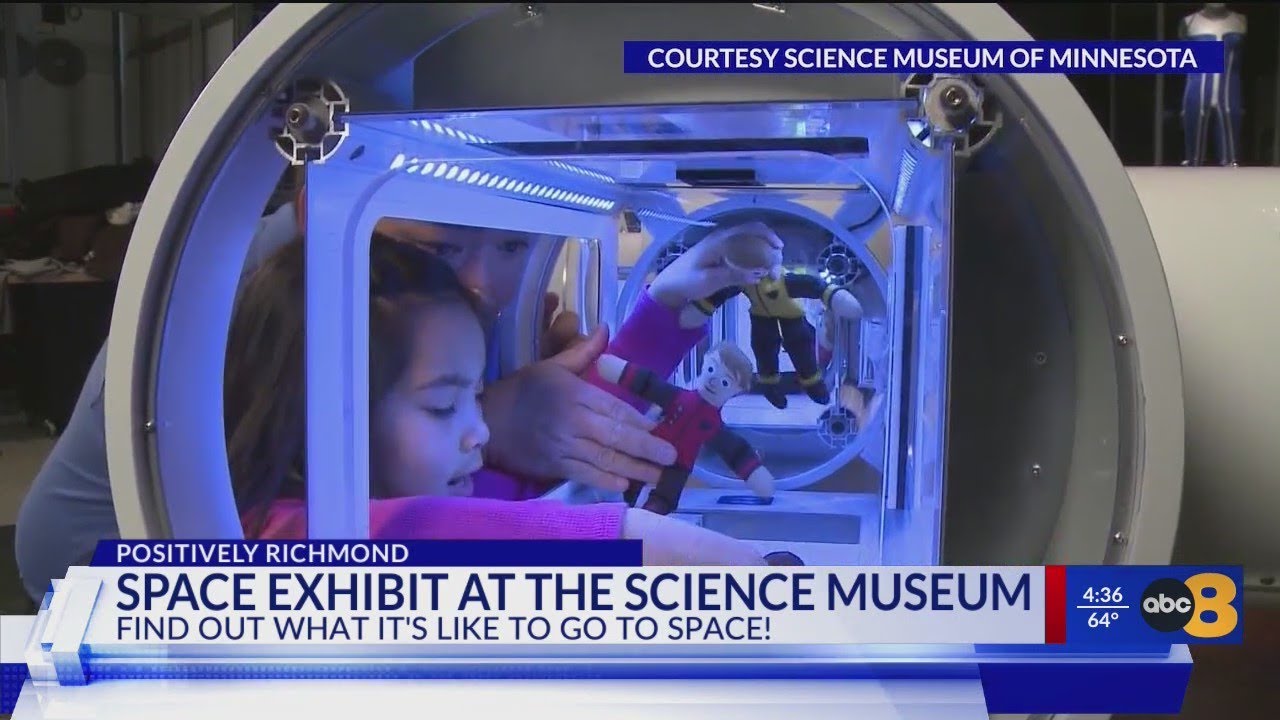The image is a detailed still from an ABC Channel 8 news broadcast, captured at 4:36 p.m. with a pleasant temperature of 64 degrees. It prominently features the ABC logo in the bottom right corner, alongside a banner that reads, "Positively Richmond Space Exhibit at the Science Museum. Find out what it's like to go to space!" At the top right, the label "Courtesy Science Museum of Minnesota" provides credit. 

The central focus of the image is a young girl and an adult engaged in what seems to be an interactive, educational activity within the museum's space exhibit. They are situated inside a circular, plastic enclosure, which effectively simulates a living space inside a spaceship. Illuminated by soft blue lights, the pair are surrounded by dolls and props that replicate the experience of living in space. The adult appears to be instructing the child, fostering both learning and exploration, highlighting the fun and educational experience offered by the exhibit.